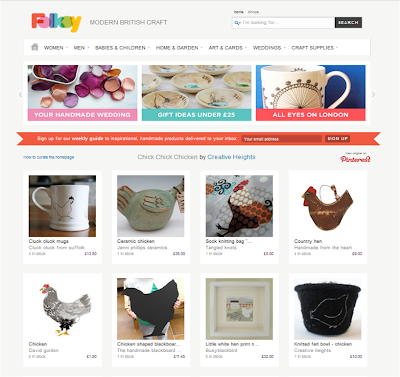The image appears to be a screenshot of a business webpage belonging to "Folksy," a modern British craft marketplace. The Folksy logo is prominently displayed in the upper left corner, and there's a search bar on the right. The main navigation bar at the top of the page includes categories such as Women, Men, Babies and Children, Home and Garden, Art and Cards, Weddings, and Craft Supplies, each featuring a drop-down menu.

Below the navigation bar are three featured images. The first image showcases purple, pink, and yellow wedding rose petals under the heading "Your Handmade Wedding." The second image highlights hand-painted bowls with the caption "Gift Ideas Under 25 Pounds." The third image features a white tea or coffee cup with a Ferris wheel design, captioned "All Eyes on London."

A horizontal orange ribbon-like stripe below these images promotes a monthly guide subscription service. It reads, "Sign Up for Our Monthly Guide as Inspirational Handmade Products Delivered to Your Inbox," with a field for entering an email address.

Further down, the page displays a range of products related to the search term "Chick Chick Chicken" by Creative Heights. These chicken and rooster-themed items include:
- A "Cluck Cluck Mug"
- A gray ceramic chicken
- A sock knitting bag adorned with a rooster, priced around three pounds
- A "Country Hen," described as a chicken in gray, white, black, yellow, and red hues
- A dark gray chicken-shaped blackboard
- A white hen print framed for wall display
- A black knitted felt bowl featuring a chicken outline

Due to the small size and blurriness of the image, specific prices for these products remain unclear. No additional text is present in the image.